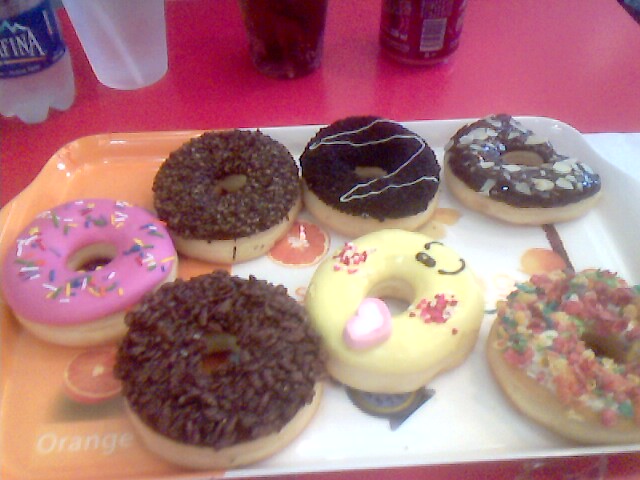The image is a detailed photograph of a tray of seven assorted donuts, each uniquely decorated, sitting on a red table. The tray, adorned with imagery of oranges and the word "orange," appears to be made of plastic. In the background, a variety of beverages can be seen, including an Aquafina water bottle, a clear plastic cup with a straw, a canned soda—likely Dr Pepper or Coca-Cola—alongside a glass filled with soda.

From right to left, the donuts are arranged as follows: the furthest right donut features a pink glaze with colorful rainbow sprinkles. Next to it, two donuts are topped with chocolate glaze and chocolate flakes; one of these also displays a zigzagging white drizzle while the other includes a smiley face and a heart-shaped candy. Further to the left, there's another chocolate-glazed donut, this time covered with coconut flakes. Conclusively, there is a plain glazed donut adorned with chunks resembling Fruity Pebbles cereal. Each donut presents a vibrant and appetizing appearance, promising a delightful experience for any sweet tooth.